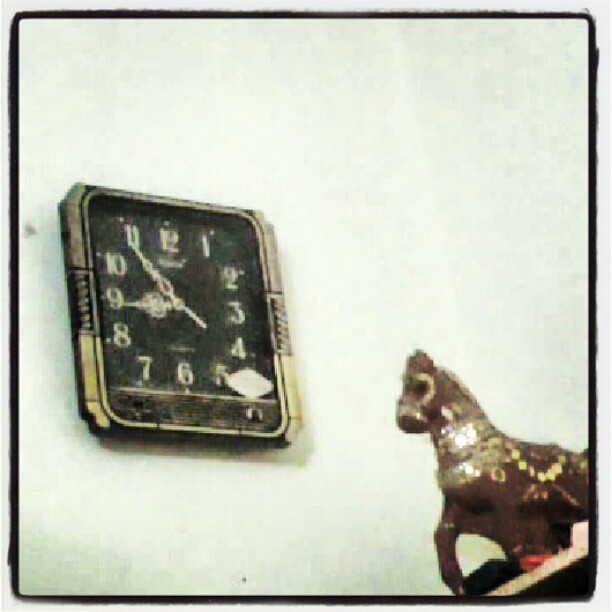This slightly out-of-focus image captures a wall-mounted clock positioned on the left-hand side. The clock displays the time as five minutes to nine and features a metallic surround with intricate, silvery ornate hands. The clock's face showcases light-colored numbers set against a dark background. Within the clock's frame, a white diamond-shaped object is also visible. To the right of the clock, sits a ceramic horse figurine adorned with elaborate tack and decorations. The dark brown horse is depicted with its right front leg raised, and it appears to be equipped with a bridle.